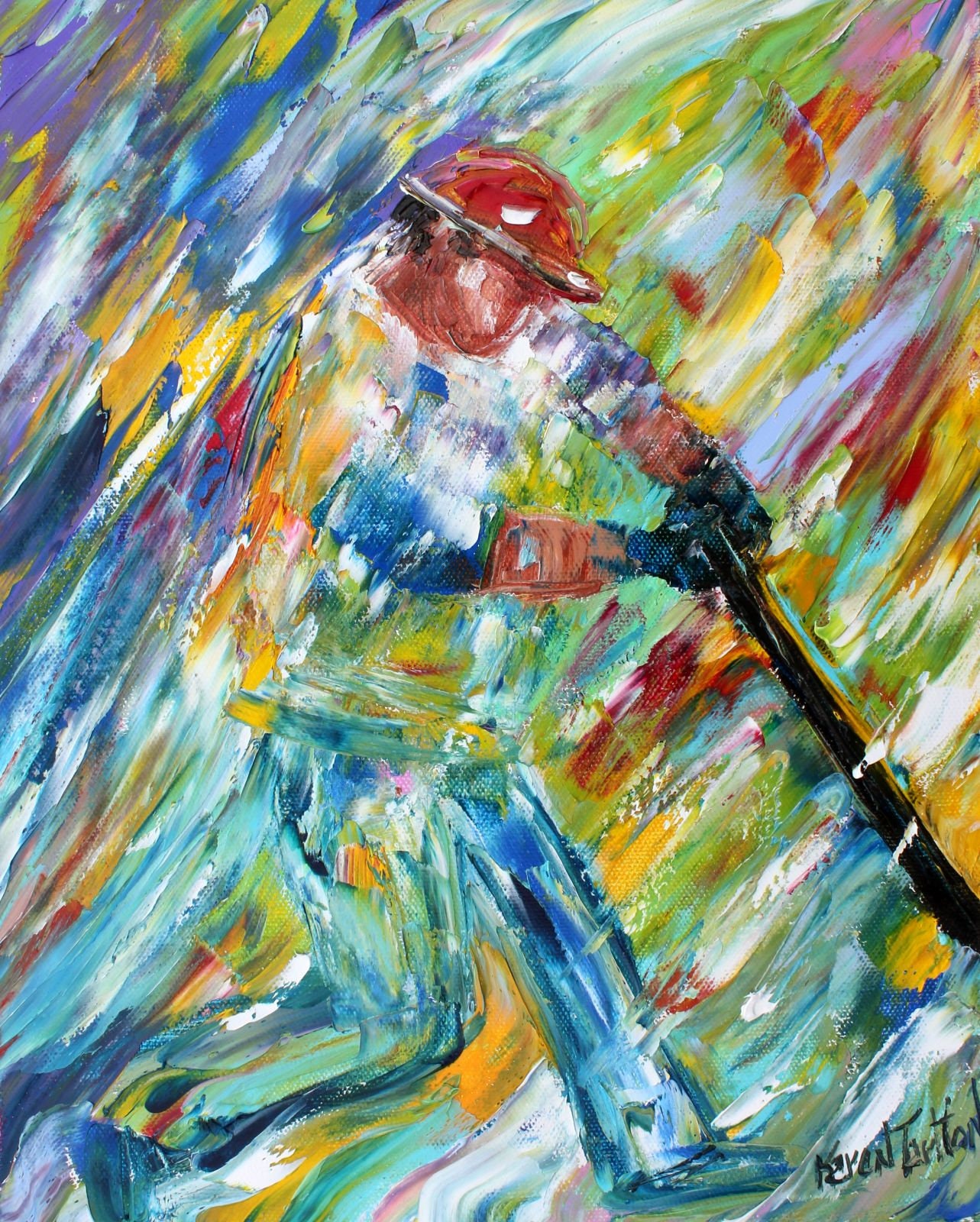The image is a detailed watercolor painting of a person, likely a baseball player, rendered with a mix of vibrant colors and abstract streaks. The figure is slightly overweight, distinguished by unique features like a red hat and reddish-black skin tone, suggesting an interplay of black and red finger paint. The player's jersey is composed of multiple colors, blending seamlessly into the background, giving the whole figure an abstract, almost ephemeral appearance. Their gloves exhibit a gradient from black palms to dark brown wrists. The pants are also multi-colored with dark blue outlines, and the shoes are darker in color, possibly black. 

The player is in mid-swing, holding a flat, black bat in their hands, with one leg forward and the other bent behind. The blending of colors like purple, green, yellow, blue, light blue, dark yellow, dark green, and dark red around the figure creates dynamic motion and depth within the artwork. The artist's signature, visible in black, is located at the bottom right corner, adding a personal touch to the expressive piece.